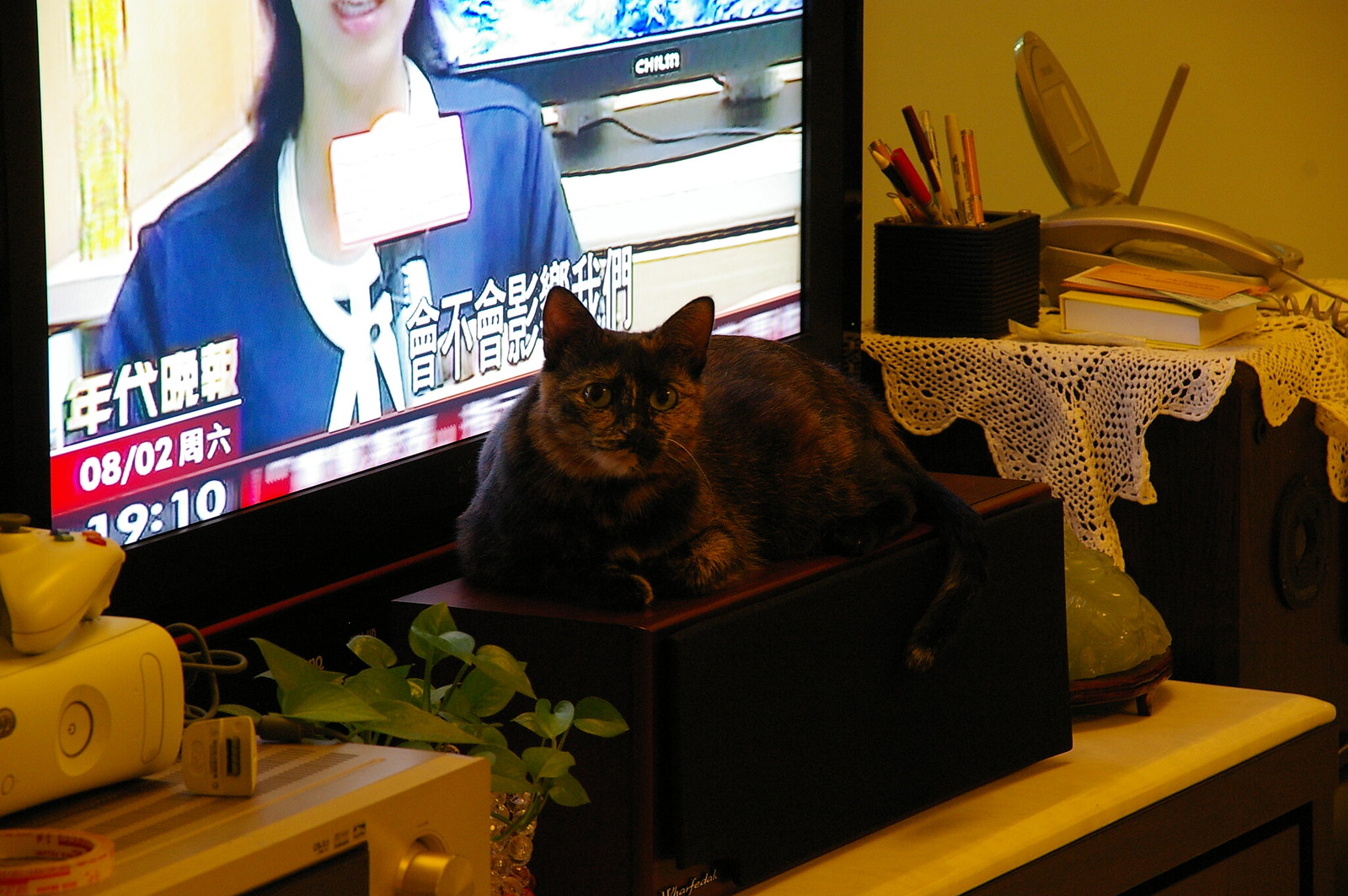In this indoor, photographic image, a cat is prominently sitting atop a brown, rectangular box, which is likely a receiver or a cable box, situated on a brown table. The feline, with a mixed dark and light brown coat and piercing green eyes, is staring directly at the camera. In the background is a flat-screen TV displaying a woman speaking into a microphone, with text in an Asian script alongside the numbers 08-02-19-10. The TV is surrounded by various items, including another receiver in the bottom left corner, topped with a white plinth. To the right, atop another table covered with a doily, there are boxes containing writing instruments, paint papers, pencils, a landline phone, and a book. The room’s walls are of an ochre or yellowish-gold muted color, adding warmth to the setting. Additionally, in front of the box on which the cat is resting, there is a small plant in a makeshift planter and another electronic device with a button, possibly a microwave or a radio, contributing to the cozy yet cluttered ambiance.